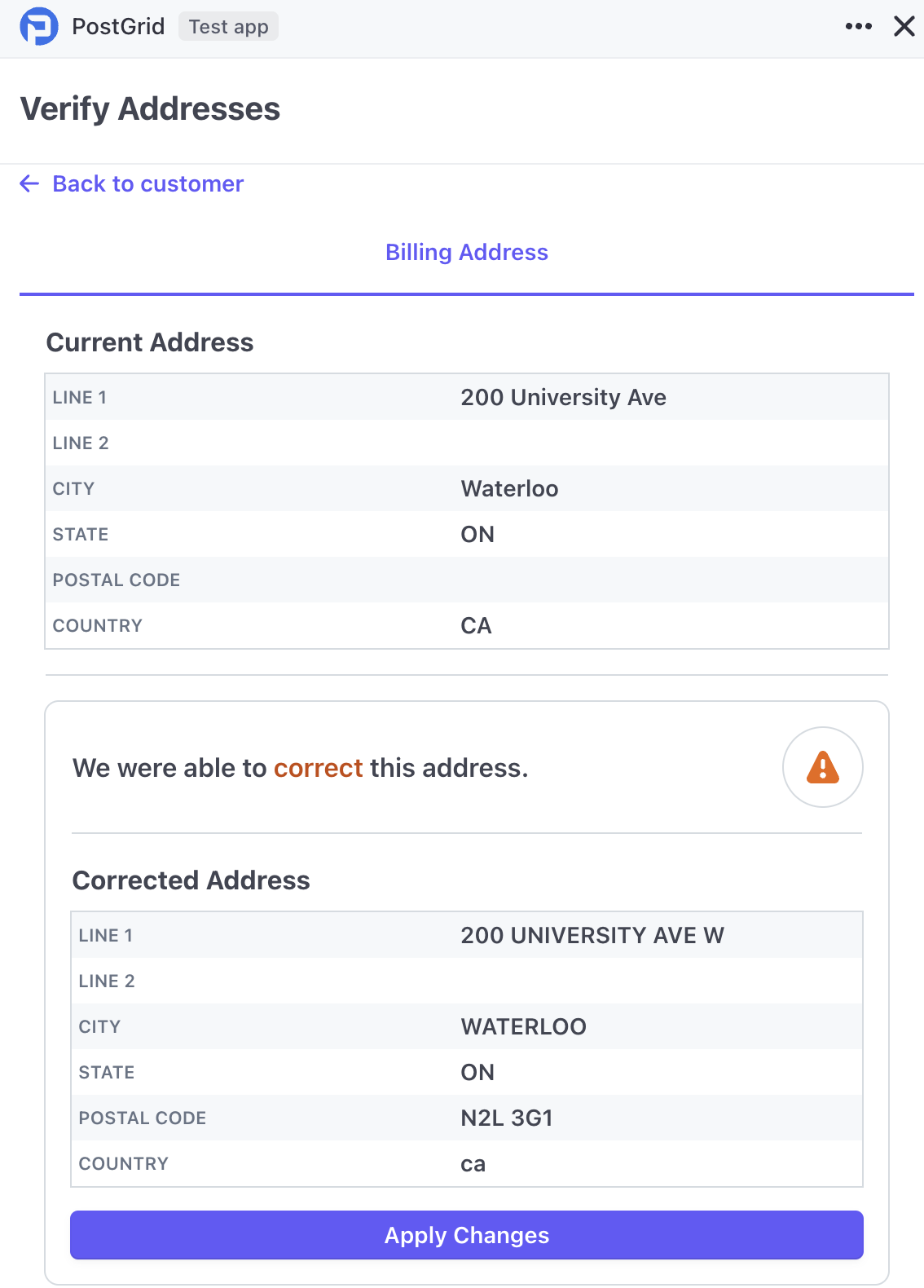This image appears to be a screenshot from a section of an application or website, specifically themed with a clean, minimalist design primarily featuring a white background and black text, with selective use of blue and purple highlights. At the top of the page, there is a header displaying a circular blue icon with a white "P" in the center. Next to this icon, the text "Post Grid" is prominently displayed, alongside the label "Test App" and a clickable "X" for closing this section.

Below the header, the text "Verify Addresses" is presented in bold black, guiding the user on the purpose of this page. Underneath, there are navigational links such as "Back to Customer" in blue or purple, and "Billing Address" highlighted in purple. The section then details "Current Address" in black text, with fields for line one, line two, city, state, and postal code listed. The current address shown is "200 University Ave, Waterloo, Ontario, Canada."

Further down, there is a notification box denoted by an orange caution sign, stating that the address has been corrected. The text "We were able to correct this address" and "Corrected Address" are also highlighted in orange. The corrected address provided is "200 University Ave W, Waterloo, Ontario, N2L 3G1, Canada."

Towards the bottom of the page, there is a prominent blue button labeled "Apply Changes," which users can click to confirm and use the corrected address. This detailed breakdown indicates that the user is interacting with the address verification section of the Post Grid application.